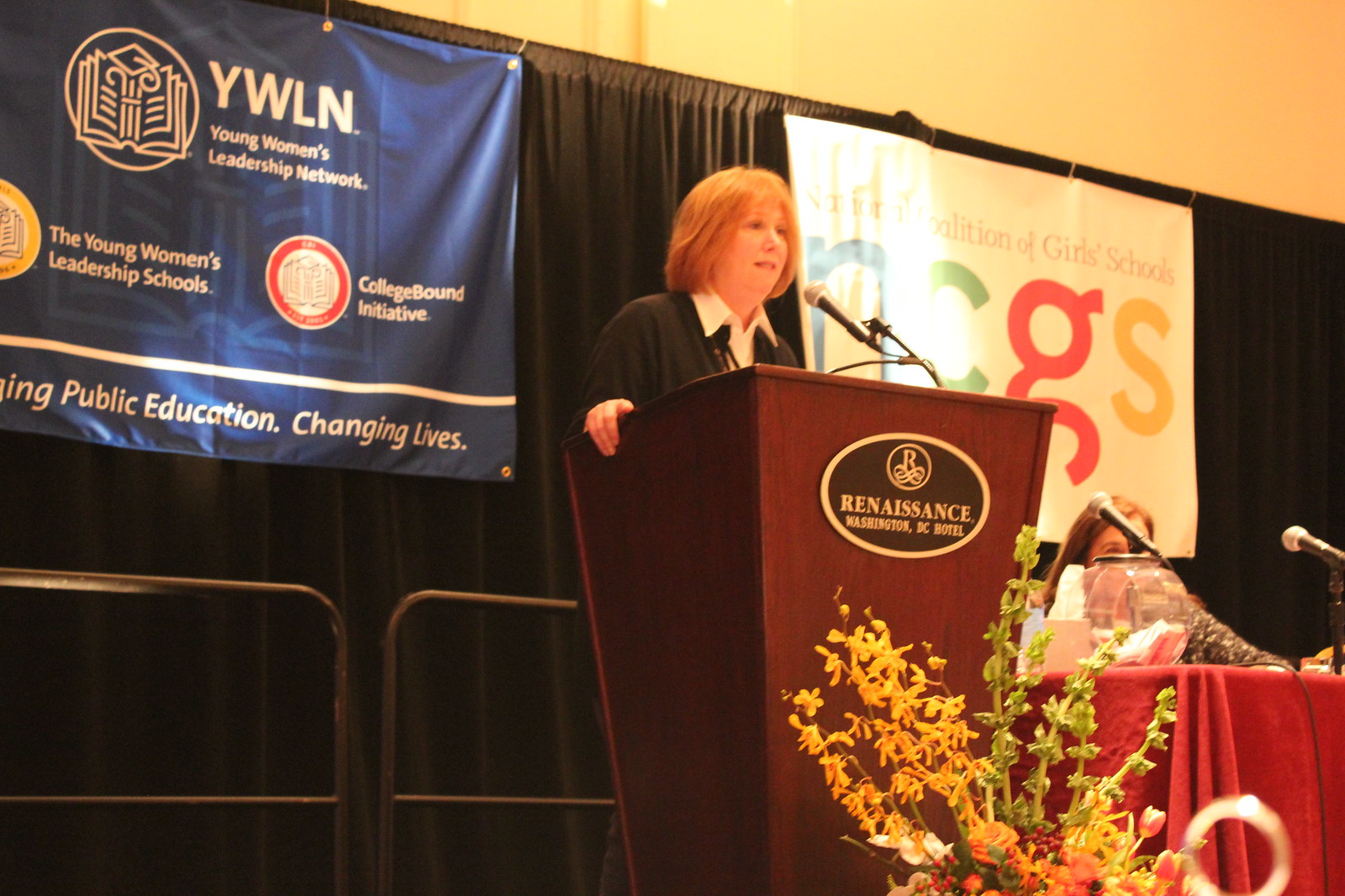In this detailed image, a woman with reddish short hair stands at the center behind a wooden podium that features a black and gold oval plaque reading "Renaissance." She grips the sides of the podium, speaking directly into a microphone. She is dressed in a white collared shirt with a black jacket. To her right, there's a table partially visible, covered with a red tablecloth, where another woman sits with microphones positioned in front of her, indicating a panel discussion or conference setting.

The backdrop consists of black curtains with two prominent banners. The left banner is blue with white lettering and a book image, displaying the text "YWLN, Young Women's Leadership Network, The Young Women's Leadership Schools, College Bound Initiative, Public Education, Changing Lives." The right banner is white with colorful letters, mentioning the "Coalition of Girls Schools, NCGS."

In the bottom right corner, yellow flowers are visible, adding a splash of color to the scene. The image is set indoors, capturing a formal event centered around public speaking and leadership within the context of the Young Women's Leadership Network. The overall ambiance is professional, with a palette that includes tan, black, blue, yellow, red, brown, gold, green, and maroon.